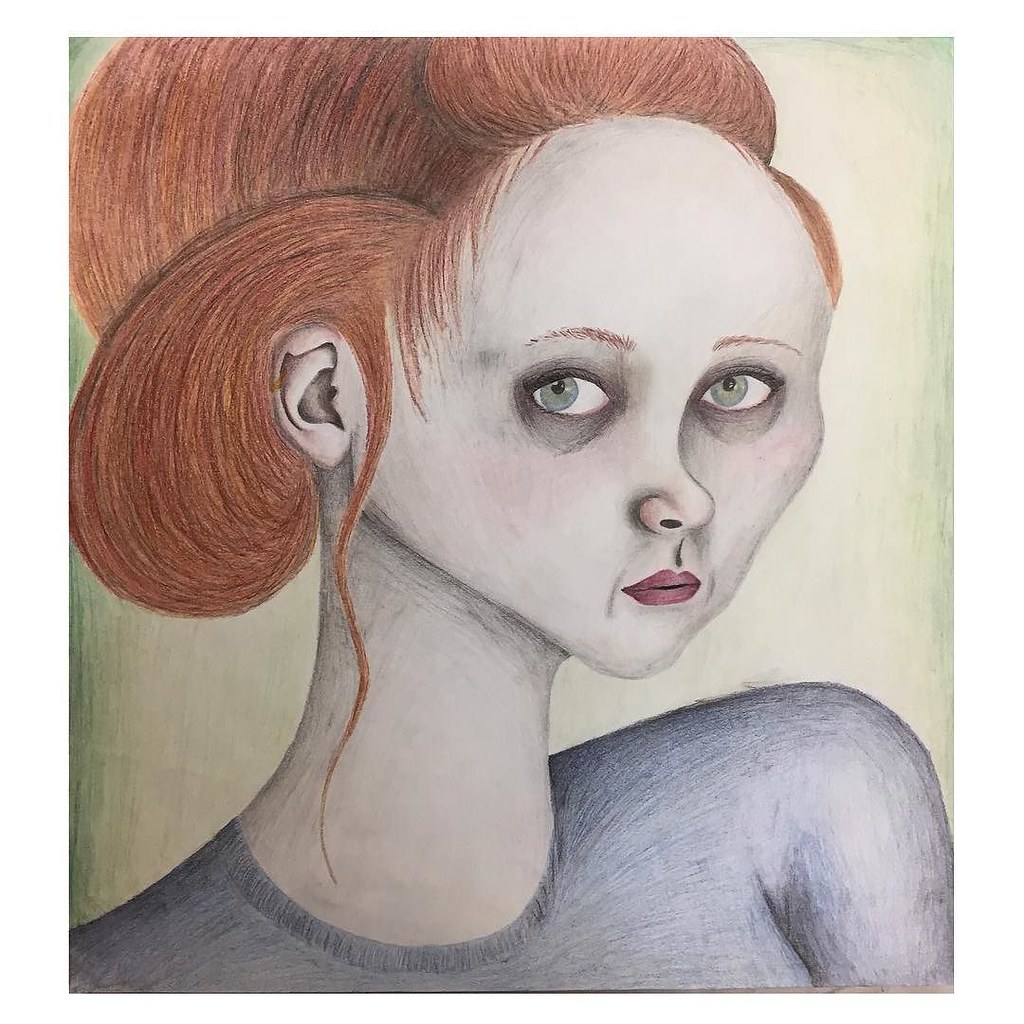The image is a contemporary abstract sketch of a woman's face set against a greenish, pea-green background that darkens towards the edges, transitioning to a lighter beige in the center. The woman has a wide, pale white face with a sharp chin, a large forehead, and reddish-brown thin eyebrows. Her green eyes are accented with dark, hollow-looking circles underneath, contributing to a tired or sad appearance. Her hair, a blend of red and brown hues, is styled in a high, poofy updo with wisps cascading around her ears and down in front. The woman's red, maroon-colored lips form a straight line, adding to her melancholic expression. Shading around her nose, mouth, and under her chin further accentuate the sullen and slightly eerie mood of the piece. She is depicted with a long, skinny neck, wearing a gray-blue sweater visible around her shoulder area, though the sleeve length is indeterminate. Her head is tilted slightly to the right, but her gaze directs to the left, adding a subtle dynamic tension to the composition.